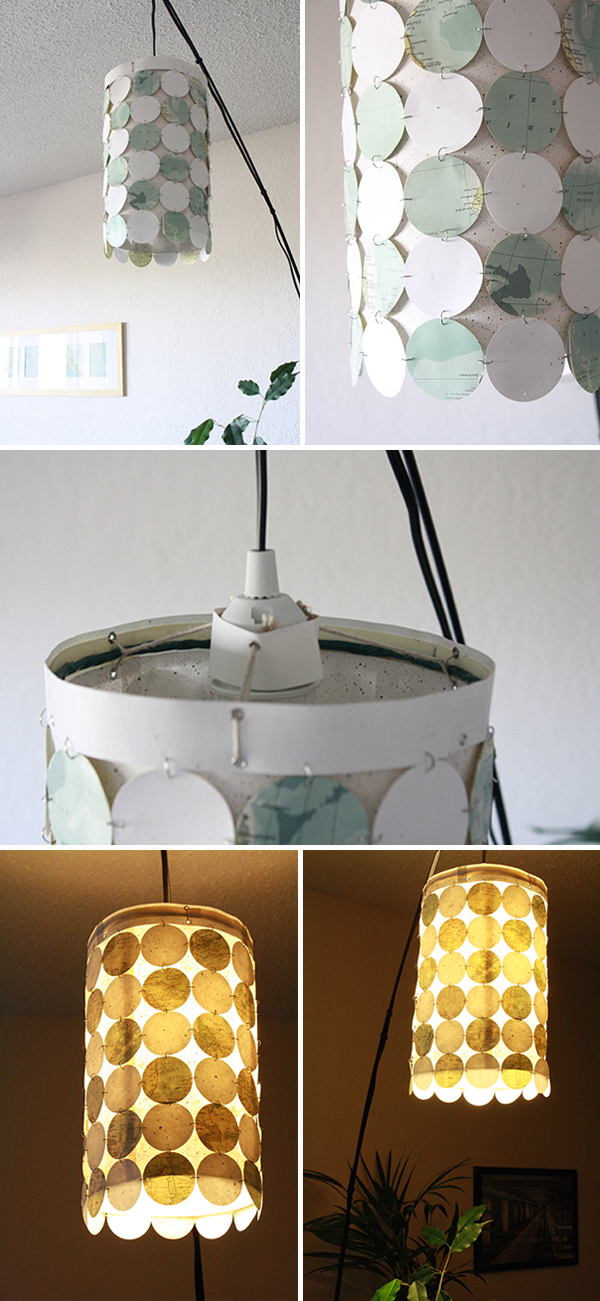This image consists of a tall rectangular collage featuring five different photographs showcasing a unique hanging lamp. The top left photo captures a full view of the lamp, made up of an array of circular pieces varying in shades of white, off-white, and green. These circles, seemingly crafted from paper or thin cardboard, are interconnected through small metal clips. The photo on the top right offers a close-up of these interconnected circles, revealing intricate details. The central photo depicts the top segment of the lamp, highlighting how it is suspended by black wires and connects directly to the light socket through a string, indicating a handmade design. The remaining two photos, positioned at the bottom, illustrate the lamp when illuminated. These images showcase its warm, ambient glow, transforming the paper-like circles into a golden hue, and also feature surrounding elements like a plant and a tree, enhancing the cozy atmosphere of the setting. The entire collage presents the lamp from various angles and states, emphasizing its craft-like construction and aesthetic appeal when lit.